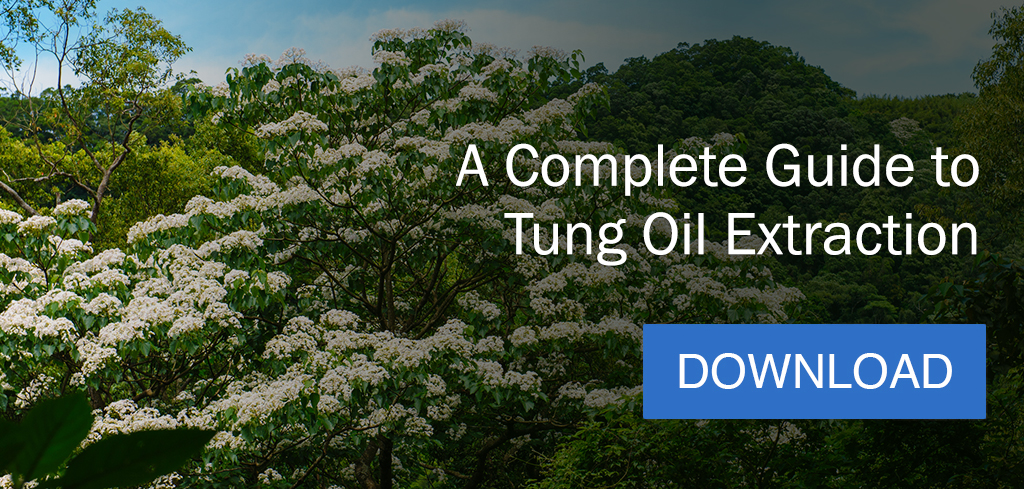This advertisement features a wide landscape photograph showcasing a natural setting with diverse vegetation. The foreground highlights slender, dark-branched trees interspersed with clusters of white flowers and green leaves. To the left of the image, there are more traditional-looking green trees, while the right side hosts bushy trees where dense foliage obscures the branches, creating a shaded, darker effect. The terrain includes a slight rise, resembling a small hill adorned with white and pink flowers. The overall image reveals a gradient sky, light blue on the left with white clouds, transitioning to a darker shade on the right.

Overlaying the right-hand side of the image, the advertisement text reads in white, "A Complete Guide to Tongue Oil Extraction," paired with a light blue rectangular button labeled "Download." This design suggests the image is likely used as a promotional banner for a website or mobile advertisement, seamlessly integrating textual information with the scenic backdrop.